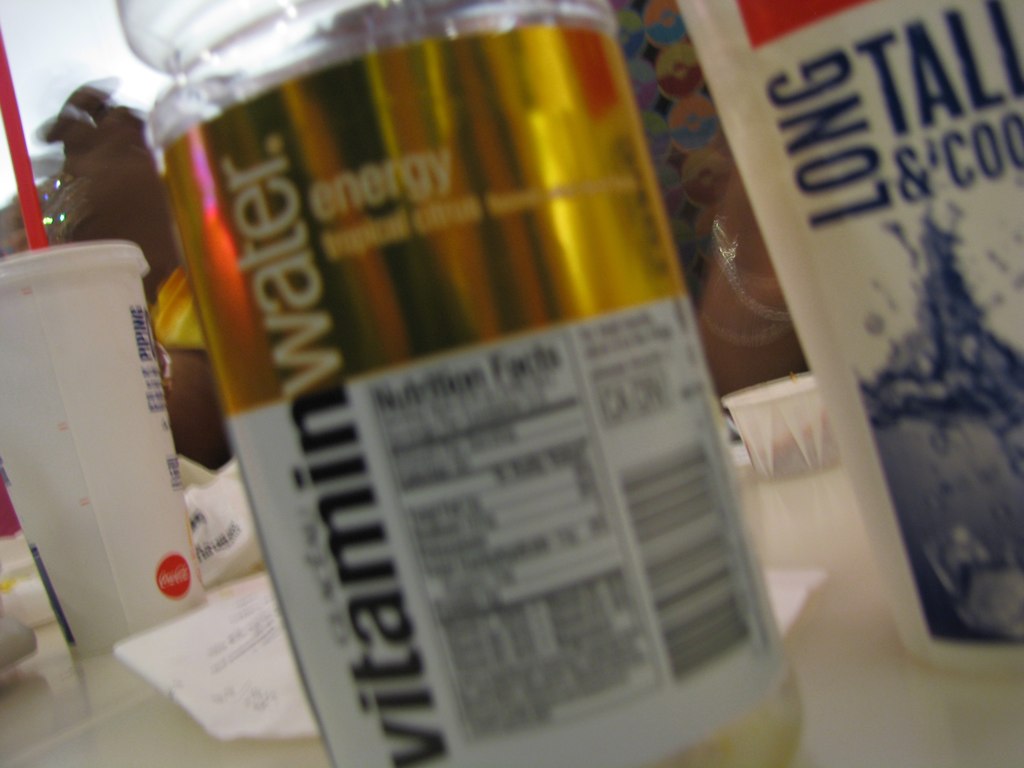The photograph captures a table at a fast-food restaurant, with a variety of items arranged on a slick tablecloth. The central focus is a bottle of vitamin water featuring a shiny gold and white label that reads "energy, tropical citrus." The label includes a section with nutrition facts, ingredients, a barcode, and California bottle deposit information. The image is blurry in the foreground, making some writing on the bottle difficult to read. To the left of the bottle, there is a white Coca-Cola cup with a plastic lid and a red straw, which has the Coca-Cola logo at its lower edge. A receipt is placed behind the vitamin water bottle. Between the drink bottle and other objects to the right, there is a small paper cup of ketchup. On the far side of the table, there are people with dark skin, one dressed in yellow and wearing a silver bracelet, though they are not the main focus and are partially obscured. The background also contains a cylindrical item with partly legible text that includes "long, tall, and cool," accompanied by an image of splashing water.